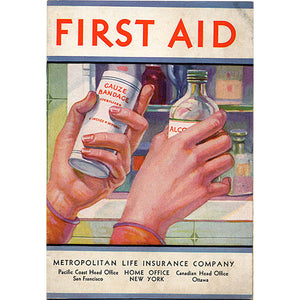The image is a vintage advertisement from the 1940s or 1950s, representing the Metropolitan Life Insurance Company. It features a colorful, illustrated scene of a medicine cabinet against a green tile wall. Two hands, one from a person wearing an orange long-sleeve shirt, are shown retrieving items from the cabinet. The left hand holds a cylindrical white canister labeled "gauze bandages," while the right hand grasps a clear glass bottle labeled "alcohol." Behind these items, the cabinet is stocked with various bottles and boxes, including a brown glass bottle, a blue bottle, and boxes colored yellow and white on the top shelf, as well as a blue box and another green bottle on the bottom shelf. The scene is framed by a cream border, with the words "First Aid" prominently displayed at the top in bold red letters. At the bottom, it reads "Metropolitan Life Insurance Company," listing offices in San Francisco, New York, and Ottawa. The overall style and the old-fashioned medical products emphasize the advertisement's historical context.